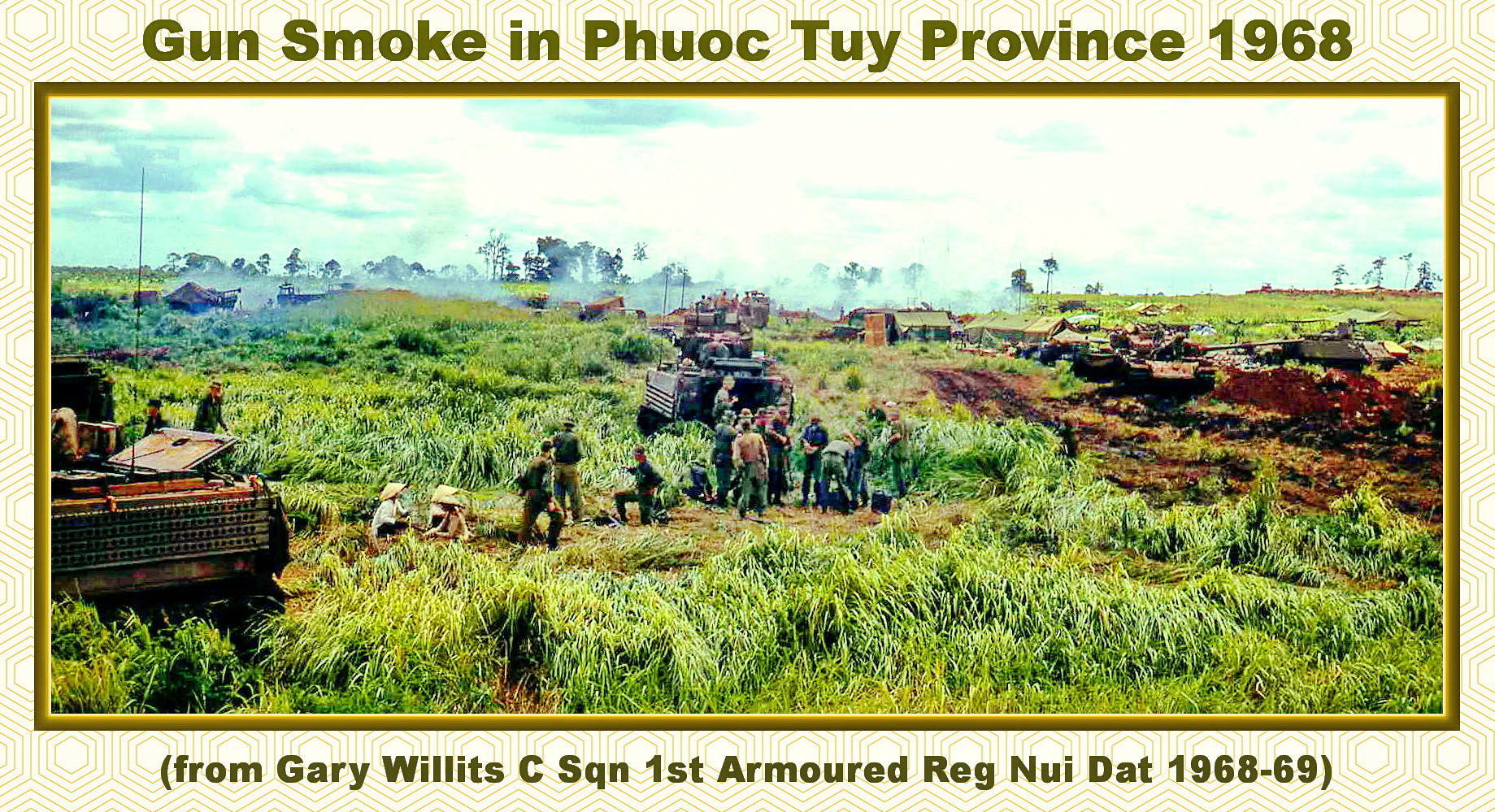The center of the image is a color photograph from 1968, bordered by a hexagonal, yellowish geometric pattern. At the top, the text in dark green reads: "Gunsmoke in Phuoc Toi Province, 1968." The bottom text, also in dark green, states: "From Gary Willits, C-Squadron, 1st Armored Regiment, Nui Dat, 1968-69." The photo captures a military scene in a Vietnamese field featuring short grass, a muddy track, and various army vehicles across the field. Central to the image is a group of soldiers with some locals in cone hats on the left side. Smoke billows in the distance, possibly from tank or artillery fire, against a backdrop of trees and a forest reaching towards the horizon.